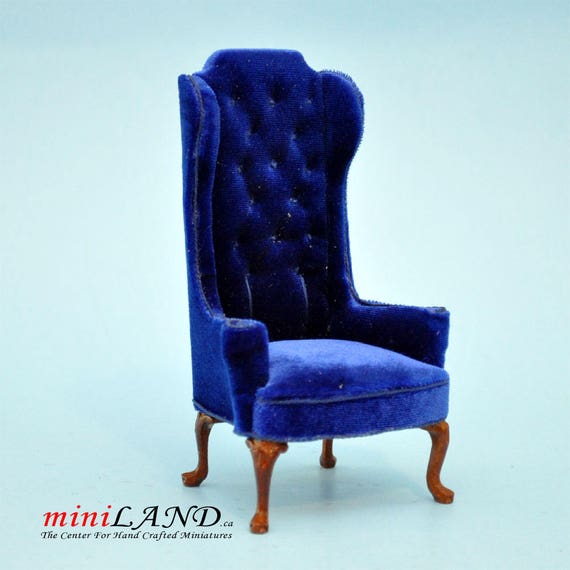The photograph showcases an expertly crafted miniature armchair set against a pale blue background. This plush, electric blue chair, reminiscent of those found in the Royal Palace in England, features a vertically elongated, tufted back, and a sleek, non-tufted seat. The chair is enclosed on the sides, forming elegant armrests that seamlessly merge into its four wooden, decorative legs that curve outward and have substantial bases.

The color palette of the image includes rich royal blue for the chair, brown for the legs, and accents in light teal for the background. Text on the image provides additional context: in red, "mini," followed by "LAND" in black, and below, "The Center for Handcrafted Miniatures," also in black. This miniature piece, positioned slightly tilted to the right, could easily be mistaken for a full-sized chair due to its intricate details and expert craftsmanship, making it a perfect addition for a dollhouse or a collector's treasure trove.